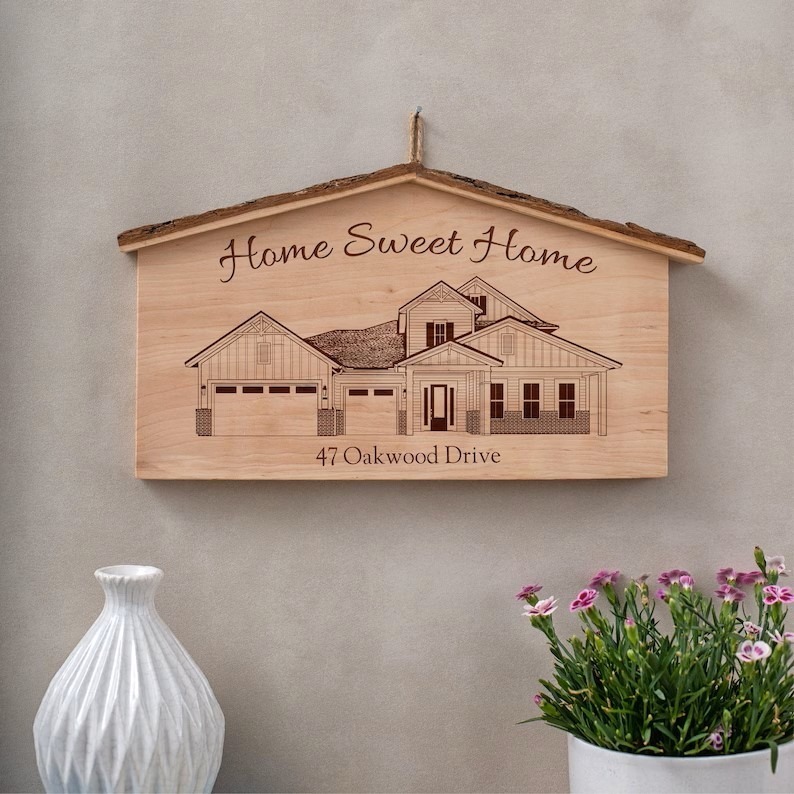The photograph depicts a wooden home decor item hanging on a purplish-gray wall. The decor piece is crafted in the shape of a house, with the top portion resembling a roof adorned with what appears to be a dark wood or bark-like texture. Intricately etched on the light wood, the words "Home Sweet Home" are prominently displayed in dark brown or black, featuring a mix of cursive and print styles for emphasis. Below the phrase, there is an illustration of a modern house with two garages and multiple windows. At the bottom, the address "47 Oakwood Drive" is centered, adding a personalized touch to the artwork. The decor piece is suspended from a nail using sinew. In the lower left corner of the image, a white ceramic vase is positioned, while the lower right corner features a white ceramic planter filled with purple flowers and green leaves.